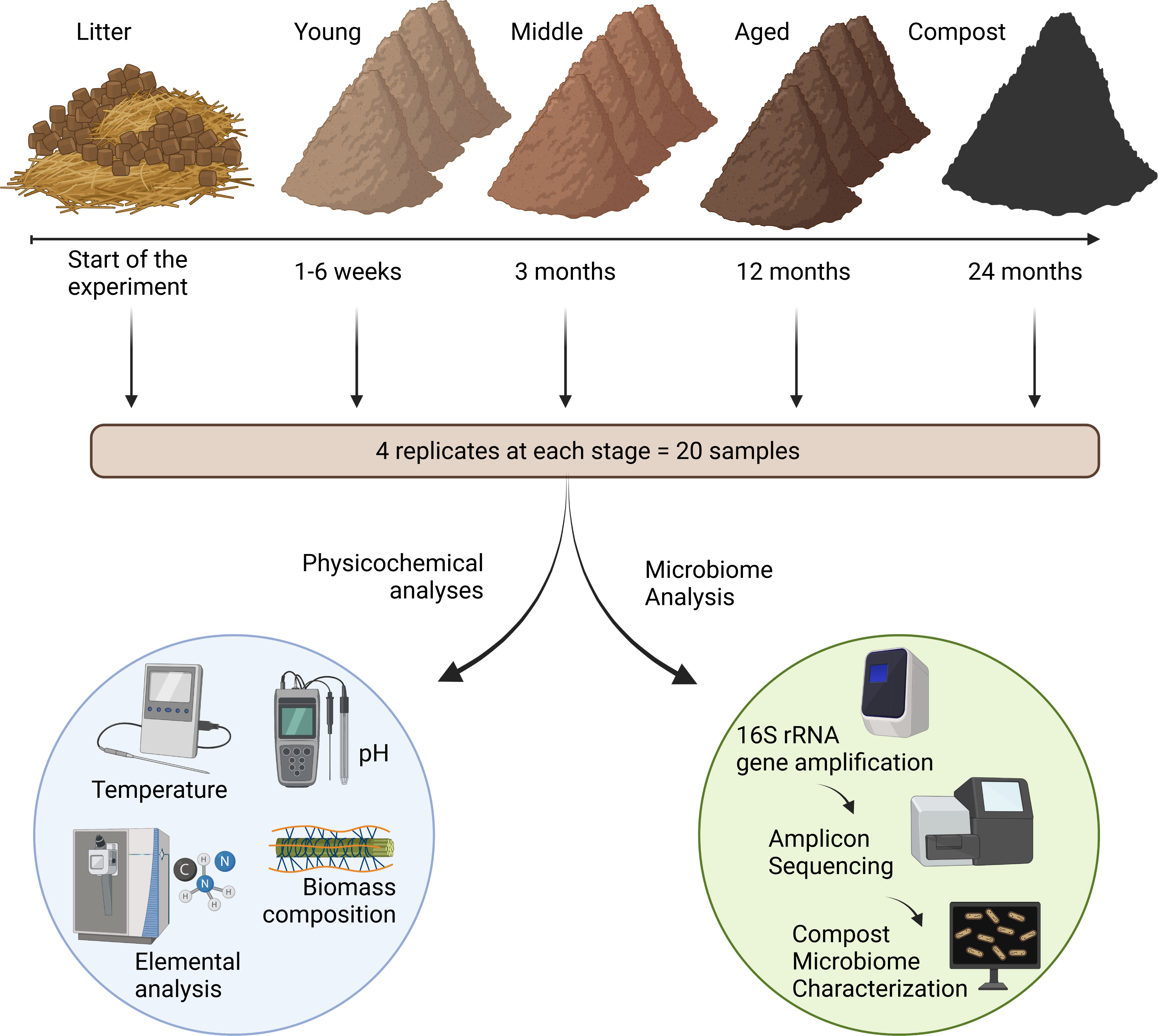The image is a scientific diagram, likely from a textbook or infographic, illustrating the composting process and corresponding analyses at different stages over 24 months. At the top, there are five labeled images showing the progression from "litter" (initial compostable materials such as green clippings, straw, and plant parts) to "young," "middle," "aged," and finally "compost." These stages are depicted from the start of the experiment through periods of 1-6 weeks, 3 months, 12 months, and 24 months, with the compost material darkening in color from a hay-like appearance to black as it matures.

Beneath these images, a tan banner notes "Four replicates at each stage equals 20 samples," indicating the sampling methodology. The diagram splits into two analysis types with labeled arrows pointing to detailed segments: "Physiochemical Analysis" and "Microbiome Analysis."

The "Physiochemical Analysis" section is represented in a light blue circle, detailing parameters such as pH, temperature, elemental analysis, and biomass composition. The "Microbiome Analysis" section is depicted in a green circle, focusing on 16S rRNA gene amplification, amplicon sequencing, and compost microbiome characterization. This extensive breakdown demonstrates the comprehensive investigation into the composting process over time.